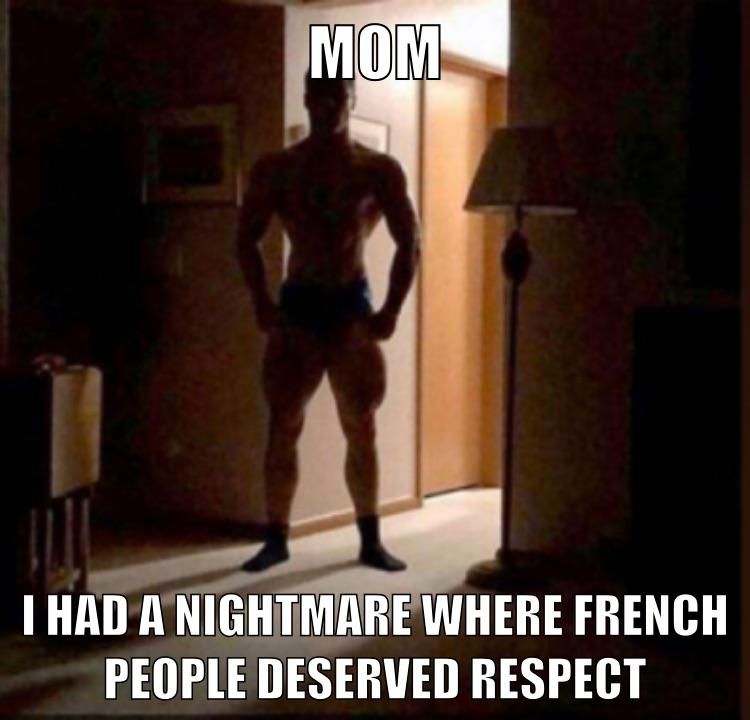The image is a meme set inside a dimly lit living room, with a muscular man standing in the middle of a backlit hallway, rendering his face indistinguishable. He is only wearing a Speedo-type underpants and socks, highlighting his impressive physique with bulging muscles. The dim room features various objects, including a lamp positioned to his right, a side table with TV trays, and framed pictures on the wall. The background reveals a creamish brown carpet and matching walls, along with wood door frames. The meme text is displayed in black outlined capital letters, with "MOM" at the top and "I had a nightmare where French people deserved respect" at the bottom, adding a comedic touch to the scene.